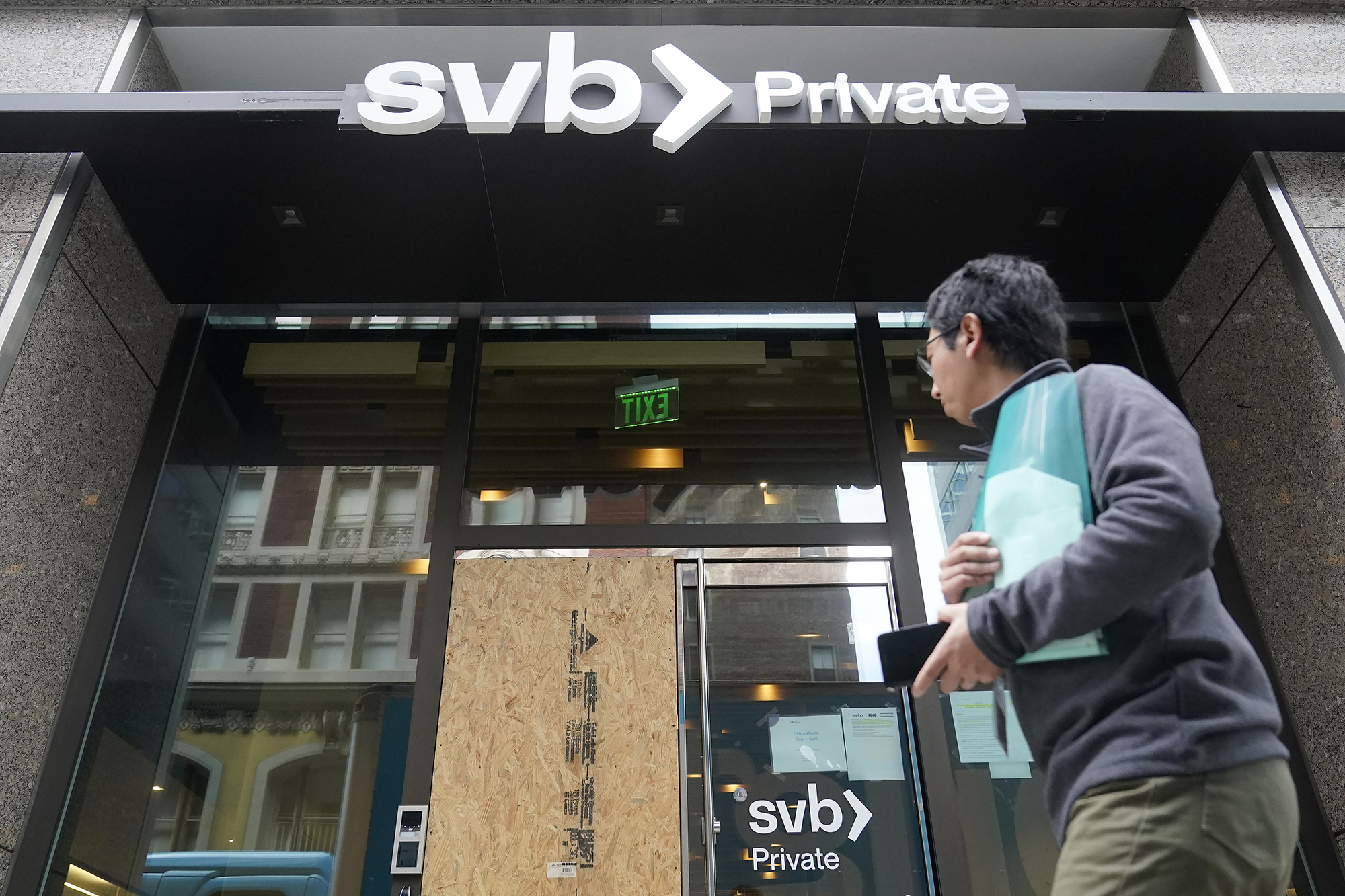The photograph captures the facade of a building, likely a bank named "SVB Private." The image is taken from a lower perspective, looking up at the structure, which features large glass windows surrounding the entrance. Prominently displayed at the top is a black horizontal beam with thick, white individual letters spelling out "svb > private." This same phrase is also visible on a decal affixed to the right glass door. The left door is notably covered by a large piece of plywood, suggesting possible recent damage. The intact right door mirrors the building's name, "SVB Private," in smaller white letters.

The glass windows provide a view into the building's interior, where a bright green exit sign and several lights are visible. Additionally, reflections on the glass reveal other nearby buildings with a mix of white, rust-colored, and yellow window frames, akin to those found in a bustling city like New York.

In the foreground, a man is walking by the entrance, looking towards the doors. He has gray and black hair, wears prescription glasses, and is dressed in a long-sleeve shirt, likely blue or grayish-purple, paired with khaki bottoms that might be shorts or pants. He holds a cell phone in his left hand and clutches a turquoise bag in the other.